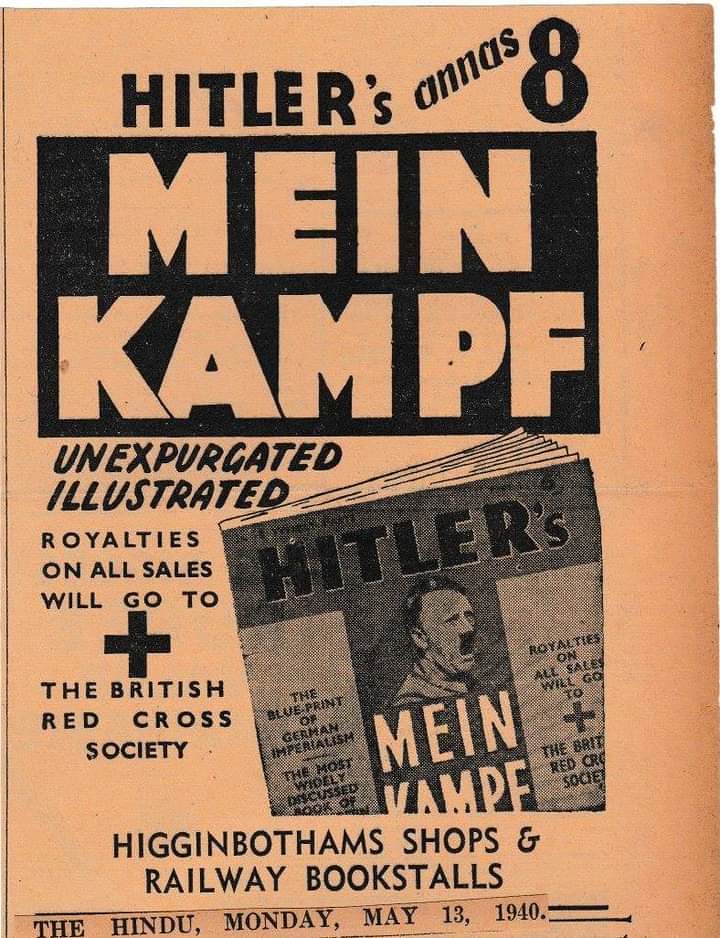The image is an aged advertisement poster with a faded peach-colored background, featuring black text. At the top, it prominently displays "Hitler's on his eighth" in bold letters. Below, there is a black rectangular box with the title "Mein Kampf" etched out in the background color. The text continues to explain that this publication is unexpurgated and illustrated, with all royalties from sales pledged to the British Red Cross Society. The poster mentions that the book is available at Higginbotham Shops and Railway Bookstalls, and references "The Hindu," dated Monday, May 13th, 1940. On the right side of the poster, there is a slightly cropped image of the book "Hitler's Mein Kampf," featuring a photo of Hitler on its cover. The advertisement combines these elements with a distinct color palette of creamsicle oranges, blacks, and grays.